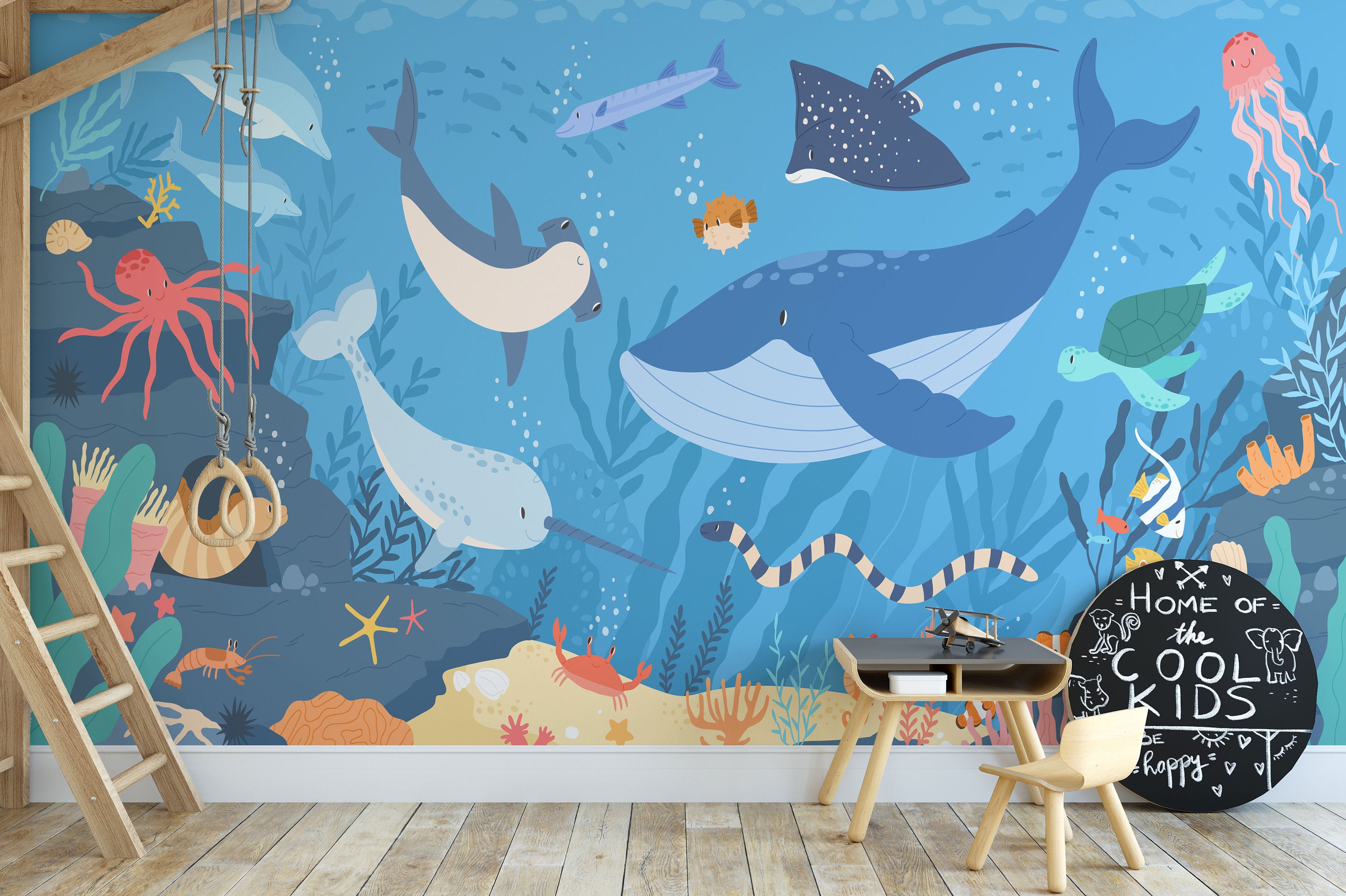This image depicts a charming small kid's room with a captivating under-sea themed mural covering the entire wall. The mural features a vast blue ocean backdrop with a brown sandy bottom, inhabited by an array of vibrant sea life. Central to the mural, a large whale gazes to the left, flanked by a hammerhead shark and a stingray. To the right of the whale, a green turtle swims, while above it, a pink jellyfish drifts. Below the whale, a narwhal and a pink octopus can be seen, adding more character to the scene. Various other marine creatures such as a shark, a crab, a starfish, a jellyfish, an octopus, some dolphins, a snake, and sea plants populate the mural, enriching the underwater ambiance.

In the foreground, a light-colored wood plank floor complements the vibrant wall art. A small wooden desk featuring an airplane and a matching wooden chair are situated towards the bottom right of the room. Leaning against the wall, a round sign with a black background and white letters declares, "Home of the Cool Kids." On the left bottom side, a wooden ladder extends upward, its destination outside the frame. White trim runs along the bottom of the mural, adding a neat finishing touch to the lively underwater scene.